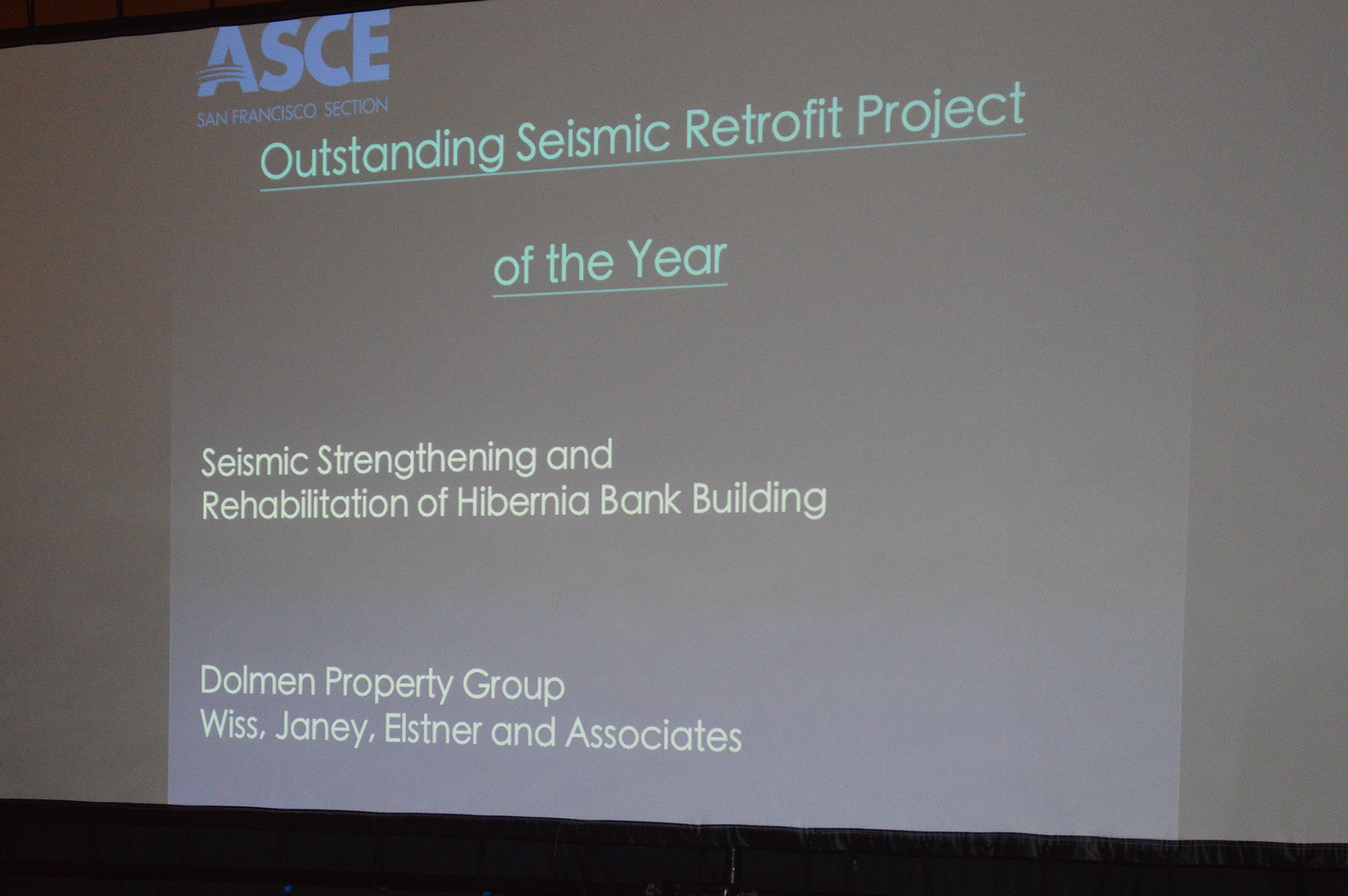The image shows a projection on a large white screen, likely in an auditorium or theater setting. The background around the screen is predominantly dark gray with areas of black at the top and bottom. In the upper left corner of the screen, in thick blue letters, it reads "ASCE," with the "A" featuring three lines. Beneath that, in smaller text, it says "San Francisco Section." Below this, in light teal or green letters, it states "Outstanding Seismic Retrofit Project of the Year," with "of the Year" underlined separately. Further down, towards the lower left of the screen, in white or light-yellow text, it says "Seismic Strengthening and Rehabilitation of Hibernia Bank Building." At the very bottom, also in white or light-yellow text, it reads "Dolman Property Group," followed by "WISS, Janey, ELSTRER & Associates." The image has darker borders on the sides, a black line that slopes downward from left to right across the bottom, and a small black triangle in the upper left corner.